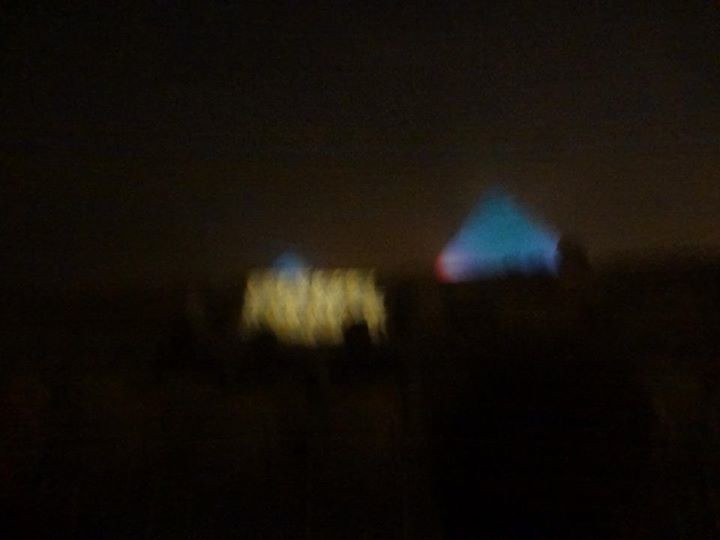This is a very blurry and dark photograph with a predominantly dark brown and black background. The bottom half is noticeably darker, with a distinct horizontal line running across the image slightly below the center. The top left side is entirely black, while the right-hand side exhibits a lighter brown hue. Dominating the middle of the image are two distinct shapes that stand out due to their brightness and contrasting colors. The left shape is a yellow rectangle adorned with some black markings and two black circles at its bottom corners. Positioned slightly to the right of the rectangle and higher up is a blue triangle with varying colors at its bottom points—black on the right and red and white on the left. These shapes might be emitting light, contributing to their noticeable presence in the otherwise dark setting, and could possibly be interpreted as light sources or flames. However, due to the image's overall blurriness, the exact nature of these objects remains unclear.